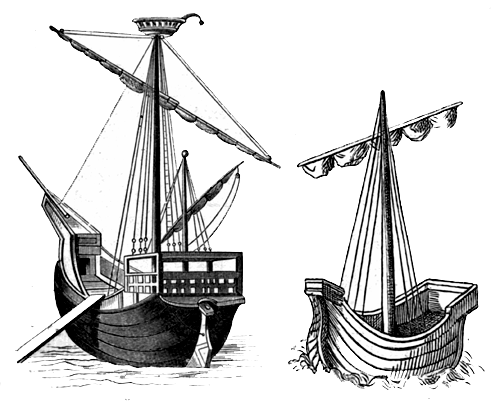The black-and-white hand-drawn illustration features two boats on the water. The smaller boat on the right is light-colored, possibly white, with one mast and ropes attached, giving it the appearance of a sailboat, although the sail seems rolled up or absent. The larger ship on the left is darker in color and displays more intricate details, including two masts and a crow’s nest atop the main mast. This ship also has a wooden plank extending from it, which might connect it to the mainland. Both vessels appear to be made of wood and resemble ancient sailing ships. The meticulous pencil drawing style captures the textures and elements vividly, emphasizing the historical and nautical theme of the scene.